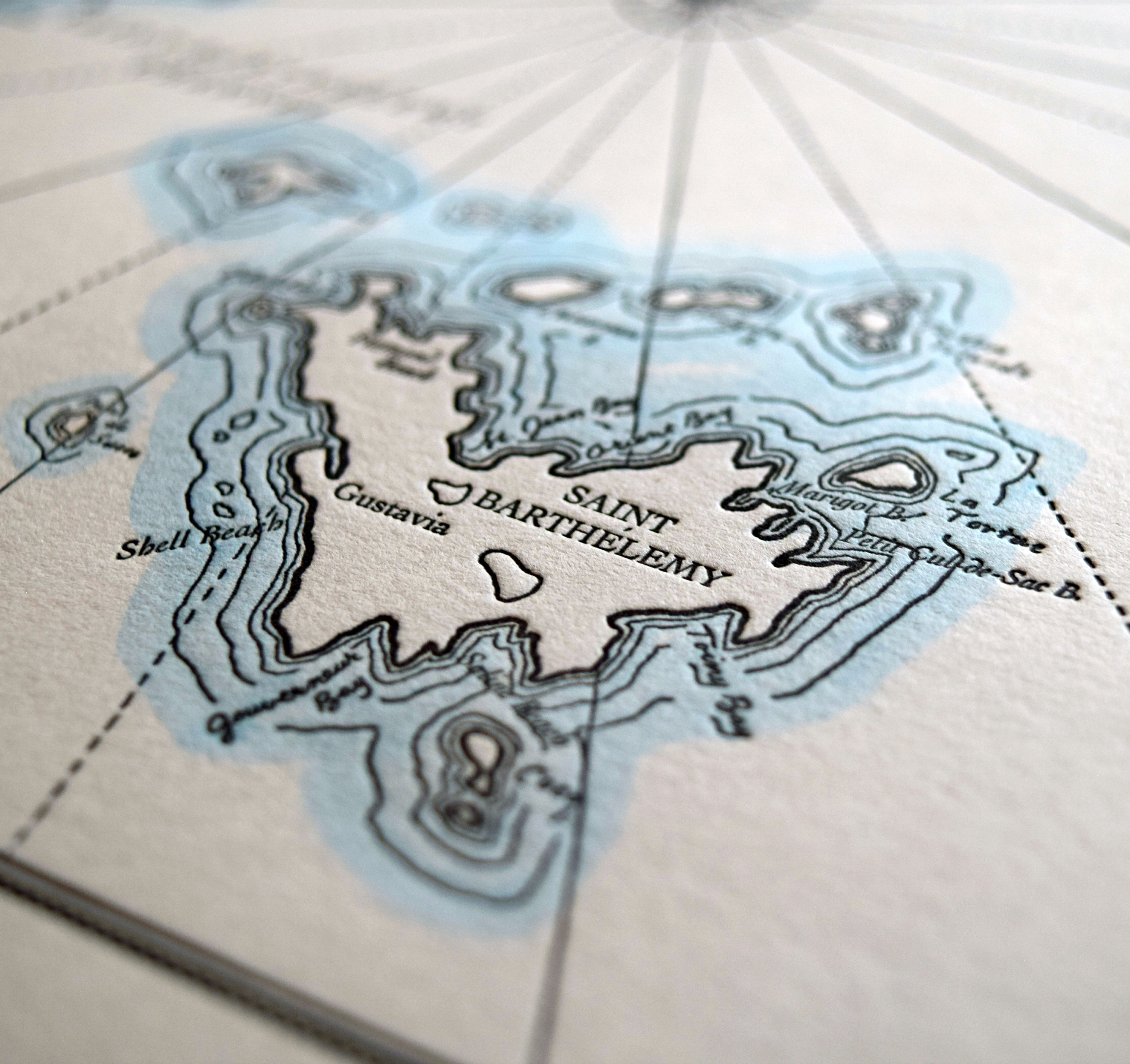The image appears to be a map focusing on the island of Saint Barthélemy, also known as St. Bartholomew, prominently labeled in a serif font. The central part of the image features this island, surrounded by light blue, likely representing the ocean. The island itself is depicted in white, delineated by a black outline. Toward the top of the image, there's a gray semicircle with rays emanating from it, potentially symbolizing the sun or another element, though its exact nature is unclear. Various locations on the island are marked, including Gustavia, La Tortue, Petite Côte d'Issac B, Marigo, and Shell Beach. Some names are in italics, some in cursive, and others in regular text, though the distinction between these styles is not specified. Above and to the left of the island, there are a few smaller, blurry islands with indiscernible names. The map features dotted lines traversing the island and segment lines resembling those on a globe, enhancing its navigational aspect.